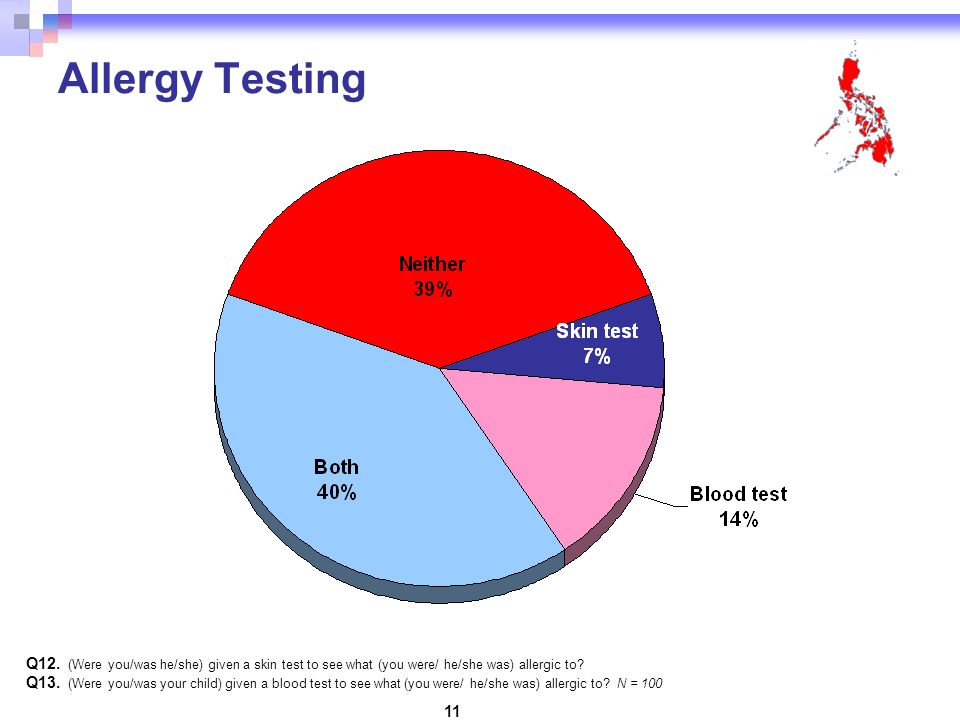The image depicts an internet page with a focus on a pie chart titled "Allergy Testing." The title is written in blue font and positioned in the upper left-hand corner of the page, which features a thin blue border along the top. In the upper right-hand corner, there is an ambiguous red shape that resembles the outline of a country or a map. At the center of the page, a large pie chart is displayed with four distinct sections. The chart's largest sections are red, labeled "Neither, 39%," and light blue, labeled "Both, 40%." There is also a smaller purple section labeled "Skin Test, 7%," and a slightly larger light purple section labeled "Blood Test, 14%." Below the pie chart, the page includes two lines of text labeled "Q12" and "Q13": Q12 asks if a skin test was administered to determine allergies, while Q13 inquires about the administration of a blood test for the same purpose, with the notation "N=100" at the end.